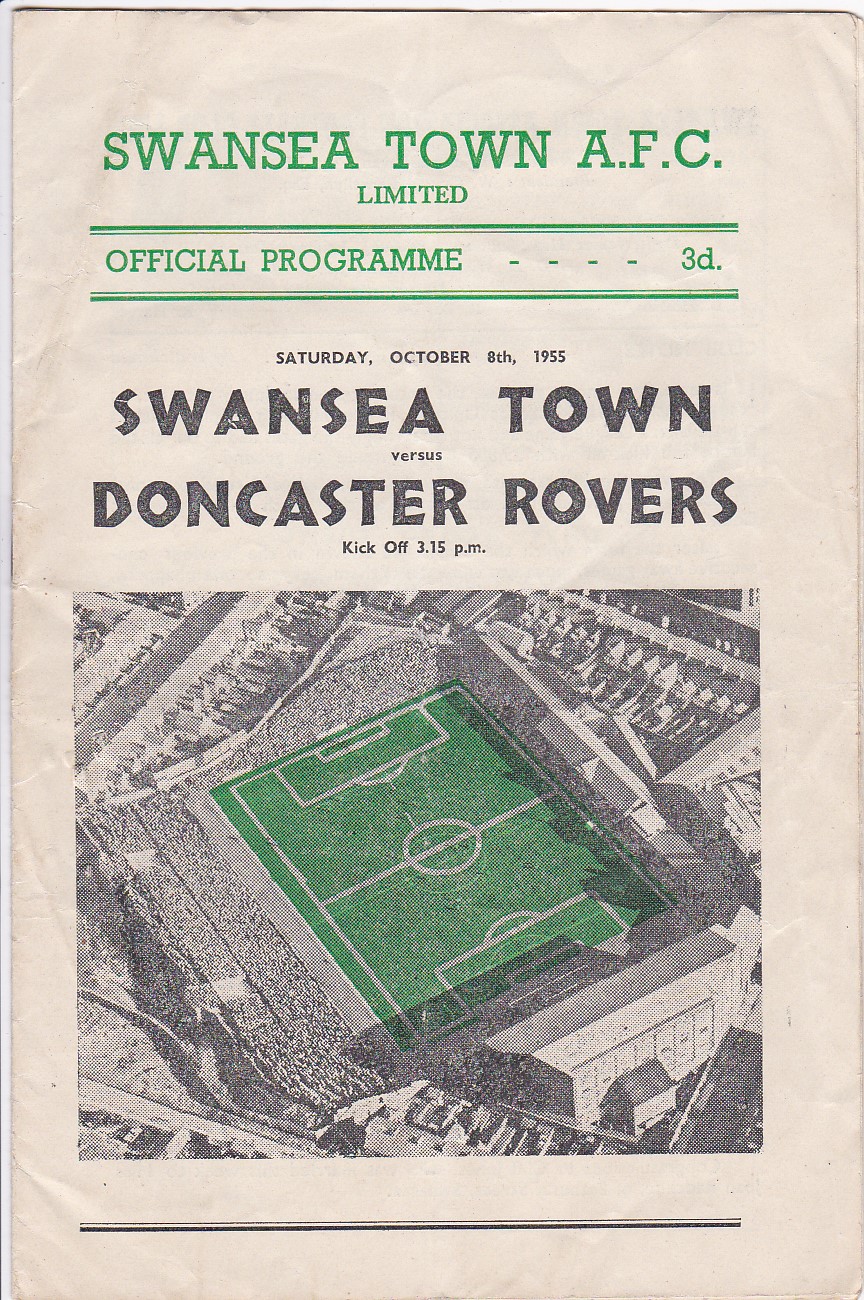This image features the cover of an official football program from almost 70 years ago, specifically for the match between Swansea Town AFC and Doncaster Rovers held on Saturday, October 8th, 1955, with a kickoff at 3:15 PM. The cover is predominantly white and shows signs of aging, appearing somewhat old and wrinkled. At the top, in green text, it reads "Swansea Town AFC Limited Official Program." Below that, in black, it lists the date and in larger letters, it announces the match between Swansea Town and Doncaster Rovers.

The focal point of the cover is a photograph that captures a view of the stadium from above. The entire image is in black and white, except for the football field, which is a vivid green with clearly visible white lines marking the field positions. The stands are filled with spectators cheering on the teams. Surrounding the stadium, there is a visible parking lot, though minimal additional details are present beyond the stadium and crowd scene. Below the photograph, a simple black line concludes the design. There are no advertisements or supplementary text, emphasizing its old-school and simplistic nature as an official program from that day.